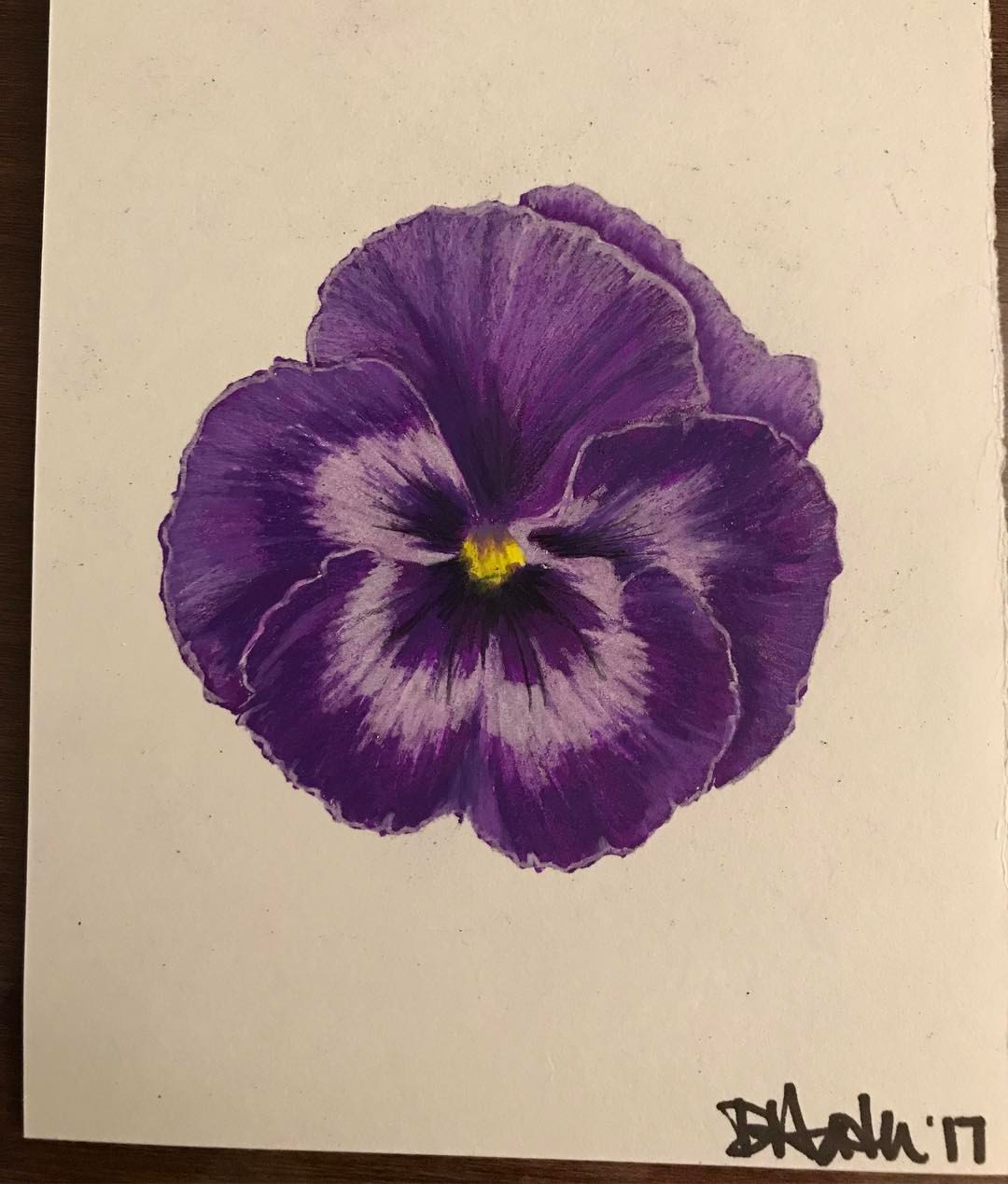This photograph showcases a vibrant piece of artwork created with colored pencils on white paper. The focal point of the drawing is a beautiful flower, resembling an orchid, with delicate purple petals. The central part of the flower features a striking yellow hue, providing a captivating contrast to the purple. Subtle lighter purple shading at the base of the petals artfully represents the play of light on the flower. The artist's signature is located in the bottom right-hand corner, although it remains indecipherable. The meticulous detailing and use of color beautifully capture the essence and elegance of this floral subject.